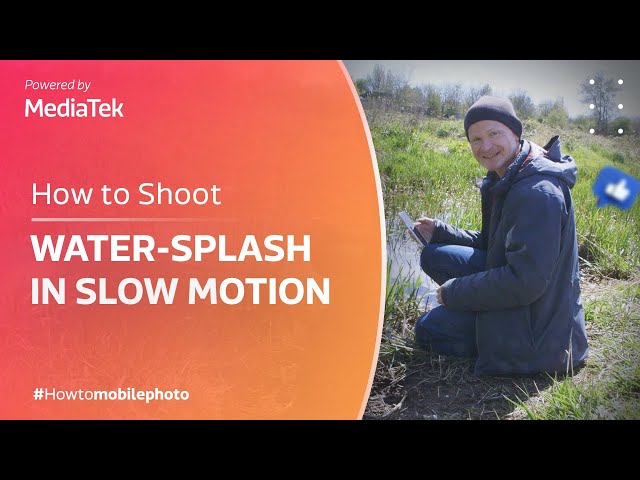The image resembles a PowerPoint slide or brochure and features two distinct sections. On the left side, a large, red-to-orange gradient circle with a white border displays in white text, "powered by MediaTek," and below it, "how to shoot water splash in slow motion." At the bottom, there's the hashtag "#howtomobilephoto." On the right side, a man is kneeling in grass next to a small puddle or pond. He’s smiling at the camera and holding what appears to be a cell phone, seemingly about to capture a photo. He is dressed in a dark knit cap, possibly black, a long-sleeve blue jacket, and blue pants. Additionally, six white dots arranged in three rows and a tilted blue word balloon with a thumbs up symbol are positioned to the upper right of him. The image itself has black borders along the top and bottom, creating a wide-framed composition.